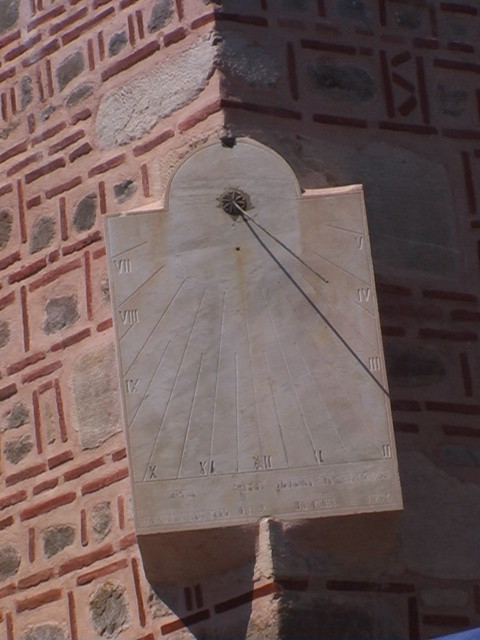This photograph captures an intricately detailed sundial, centrally positioned against a vibrant brick backdrop. The main colors in the image range from earthy tan and rich pink to a rusty terracotta, interspersed with touches of white and gray. Natural sunlight illuminates the left side of the sundial while the right side remains cloaked in shade, creating a striking contrast.

The sundial, depicted in a warm tan hue, features a prominent needle affixed towards its upper half. Roman numerals encircle the sundial's surface, with the shadow cast by the needle falling three numerals from the top, indicating the time. The sundial is meticulously placed atop a brick background with vibrant colors—a salmon pink outline and rusty terracotta red lines intricately woven together, highlighted by occasional gray tones.

This vividly detailed outdoor scene marries the timeless functionality of the sundial with the dynamic interplay of light and shadow, all set against a backdrop that enhances the visual warmth and texture of the composition.